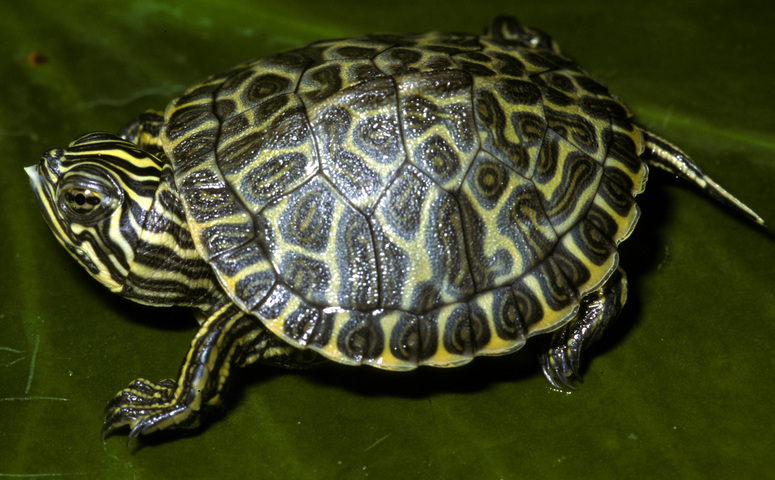In this rectangular image, which is wider than it is tall, a turtle stands prominently as the central and only object. The background features a green surface that appears slightly out of focus, resembling a large leaf or other green material. The turtle, primarily yellow with intricate darker yellow and black wavy stripes, is oriented toward the left side of the image while its tail extends close to the right edge. The head of the turtle, positioned markedly with a slightly atypical, non-perfectly round shape, features a big bulgy eye. The turtle's legs display similar coloration and striping as its head and shell, with the front leg tucked in next to the head and the back leg stretched out onto the green surface. This realistic photograph captures the turtle in vivid detail, presenting a lifelike 3D effect that emphasizes the complex patterns and colors on the turtle's shell and skin.